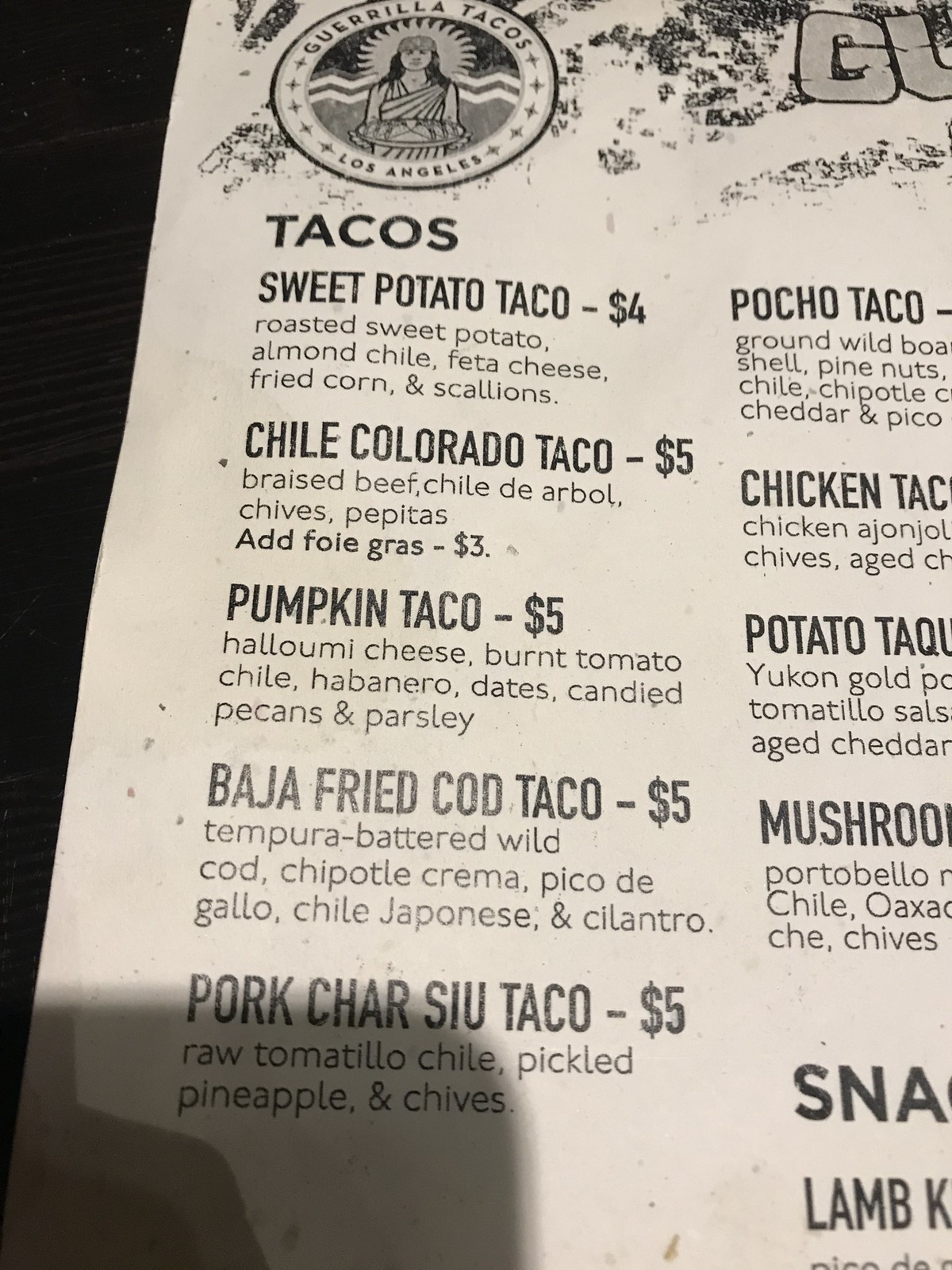**Caption:** 

_In this black and white vertical photograph, a partial view of a paper menu from Gorilla Tacos in Los Angeles is visible. The menu appears to be shot vertically, likely with a cell phone, capturing only a portion of the offerings. At the top of the menu, the name "Gorilla Tacos" and a logo featuring an image of a person with a head covering, possibly the restaurant's mascot, holding a plate of tacos, is prominently displayed. Among the readable items listed are several taco varieties: Sweet Potato Tacos priced at $4, Chili Colorado Tacos at $5, Pumpkin Tacos also at $5, Baja Fried Cod Tacos for $5, and Pork Char Siu Tacos at $5. The menu continues beyond the frame, with additional items that are not discernible in this shot._